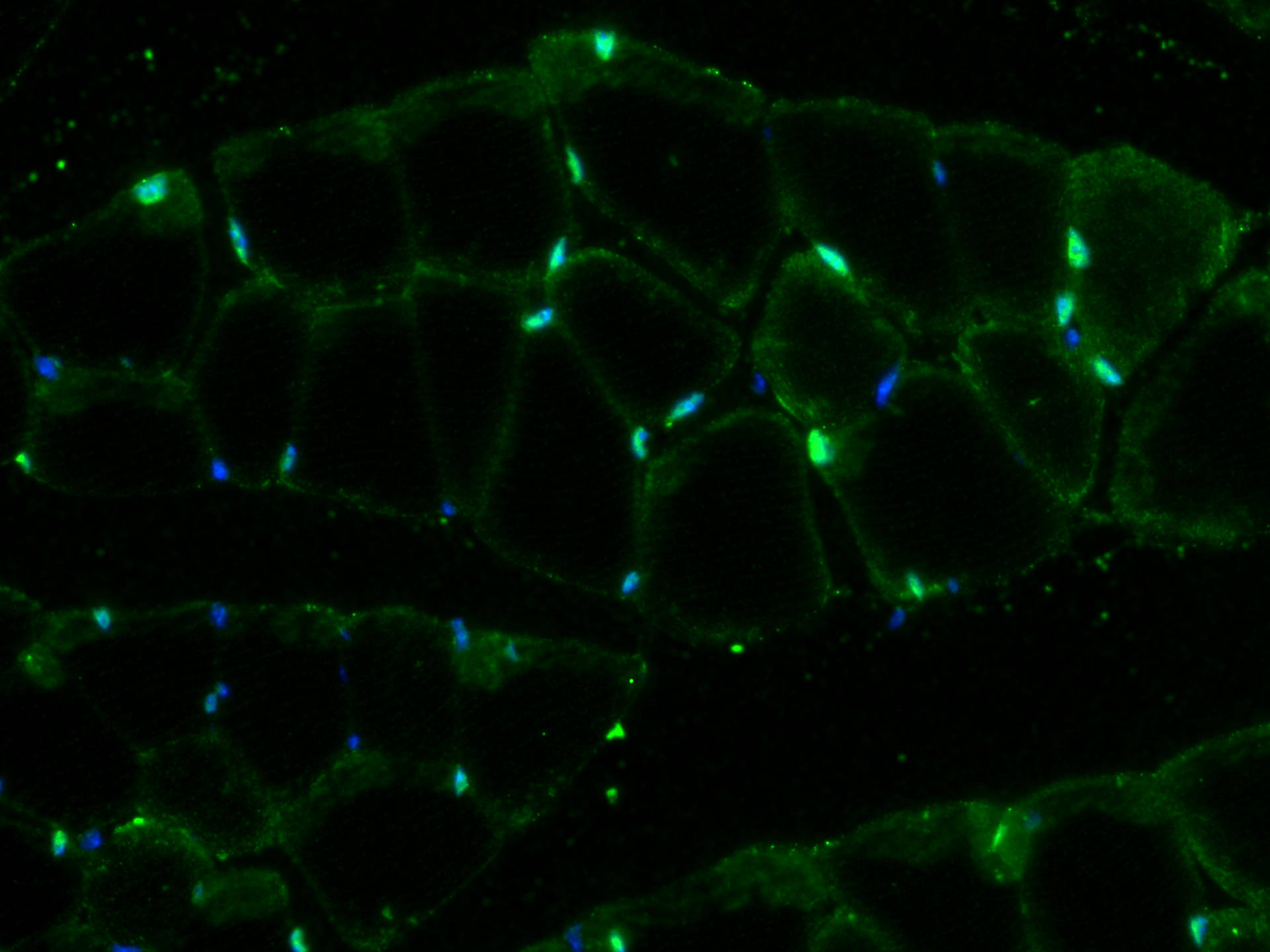The image is a rectangular landscape, approximately 30% wider than it is high, showcasing a dark, perhaps outer-space-like background. The foreground features an intricate and mesmerizing pattern of irregularly shaped, green-bordered cells that almost appear to be made of glass due to their shiny, hollow structure. These cells are grouped together in clusters, forming a larger, connected mosaic with black spaces filling the gaps between them. Each cell is outlined in bold, vibrant green, with bright green and occasional blue highlights that illuminate parts of their edges. The green lights vividly outline and border each cell, making the shapes appear distinct and almost three-dimensional. Bright green spots punctuate the cells’ corners and edges, adding to their striking, otherworldly appearance. Overall, the image exudes a sense of depth and complexity, with the prominent colors being green, blue, and black.